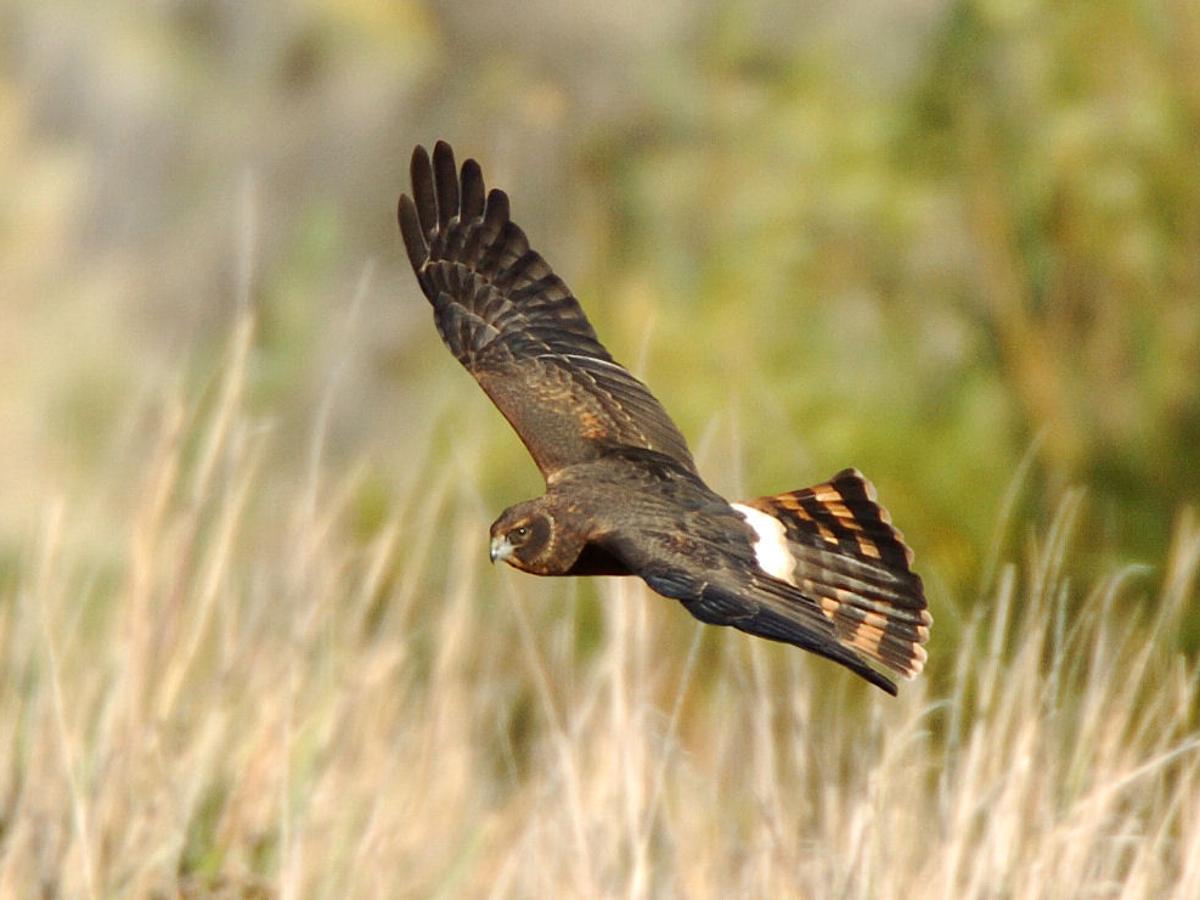In this detailed outdoor photograph, a majestic northern harrier is captured in mid-flight, gliding over a field of tall yellowing weeds and dried grasses. The bird is centered and crisply in focus against a blurred background that hints at some distant green trees. The harrier's wings are fully extended, showcasing a striking array of feathers that transition from dark brown near the body to darker hues towards the tips. Its face and body are predominantly dark brown, with lighter, almost orange-brown highlights around the eyes, adding intricate details to its piercing gaze. Notably, the bird has a small, hooked beak, which appears light gray with a darker black tip. Its tail feathers exhibit a distinctive pattern, starting with white at the base, transitioning to brown in the middle, and featuring orange stripes that culminate in orange tips at the edges. The harrier appears to be on the hunt, descending with precision and grace over the blurred grassy expanse, embodying the sheer beauty and intensity of a bird of prey in action.